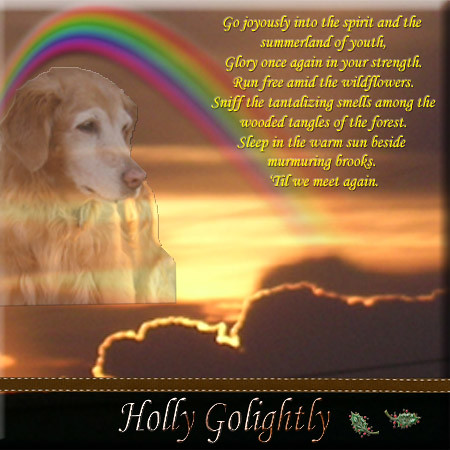This detailed tribute to the recently deceased dog, Holly Golightly, features a poignant and illustrative composite image. Dominated by a sunset with clouds and an illustrated rainbow arching from the horizon, the scene is imbued with warm brown and gold hues. Superimposed prominently within the square, beveled-edge image is a touching portrayal of Holly, likely a golden retriever, who gazes pensively. The background includes a heartfelt poem in elegant yellow lettering, reading: "Go joyously into the spirit and the summerland of youth. Glory once again in your strength. Run free amid the wildflowers. Let the tantalizing smells among the wooded tangles of the forest. Sleep in the warm sun beside murmuring brooks till we meet again." This somber yet beautiful memorial is underscored by a black banner at the bottom of the image, bearing the inscription "Holly Golightly."